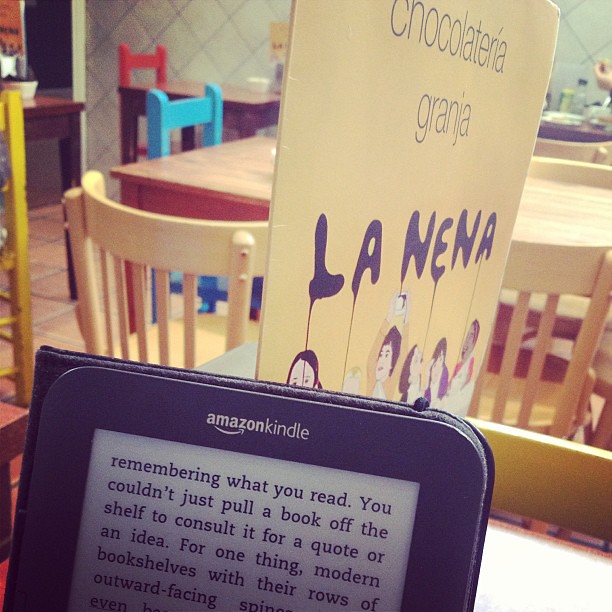In this image, we appear to be in an indoor setting, either a kitchen or a classroom for small children. Dominating the center of the image is a sign that reads "Chocolateria Granja La Nina," indicating a focal point. Just below the sign, young children are playing, suggesting a lively and active environment. 

In the bottom left corner of the image, there is a tablet device, specifically an Amazon Kindle, that displays text beginning with "Remembering what you read. You couldn't just pull a book off the shelf to consult it for a quote or an idea. For one thing, modern bookshelves with their rows of outward-facing spines...," trailing off mid-sentence.

The furnishings in the room include small, multicolored tables and chairs in hues of natural wood, blue, and red, emphasizing a space designed for comfort and activity. Scattered throughout the image are various objects and colors, including tan, purple, yellow, light blue, red, brown, and gray, adding to the room's vibrant and dynamic atmosphere. The exact time of day is unclear, but the overall scene suggests a cheerful and engaging setting for young children.